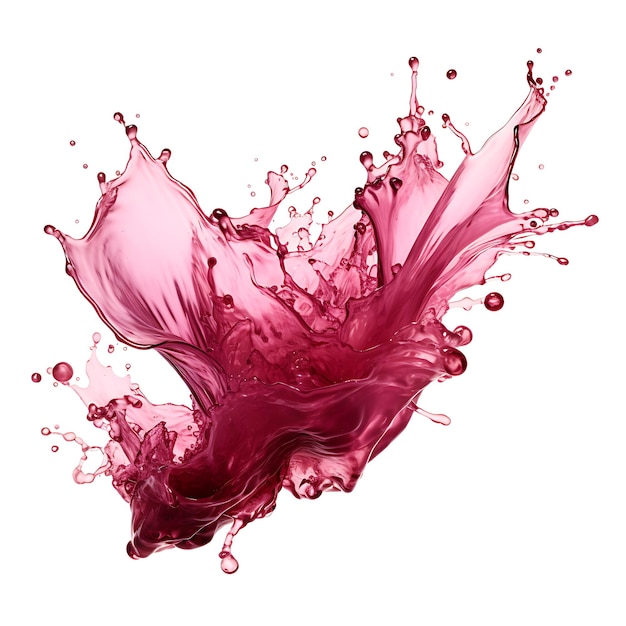This image showcases a dynamic splash of dark red to pink liquid against a white background with no borders or text. The splash appears thicker and denser at the bottom, especially in the lower left, where the color is a deeper, almost fuchsia red. Drips and droplets extend from this dense area in various directions, primarily downward and to the left, appearing as lighter pink. As the splash spreads upward toward the upper left and upper right, the liquid thins out and shifts to a lighter pink hue, with numerous tiny droplets and splatters dispersed in all directions. The overall composition is fluid and nonlinear, with a natural, organic feel, almost as if the liquid momentarily lost its container and is captured in mid-air, poised to fall.